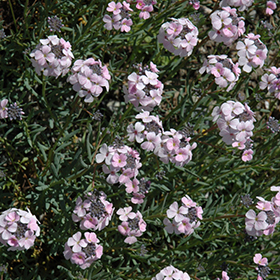The image showcases a grassy field adorned with a mixture of small flowers. These flowers primarily exhibit hues of pink, lavender, and light purple, with a few yellow ones scattered about. The grass is dark green and sparse enough to reveal patches of brown dirt underneath. The flowers, numbering around 20, form circular clusters that give an impression of spherical shapes. While the centers of the flowers are not prominently visible, some seem to show a dark gray seed-like core. This overhead shot captures a small, focused section of the field, emphasizing the delicate and colorful contrast between the flowers and the lush, shredded grass.